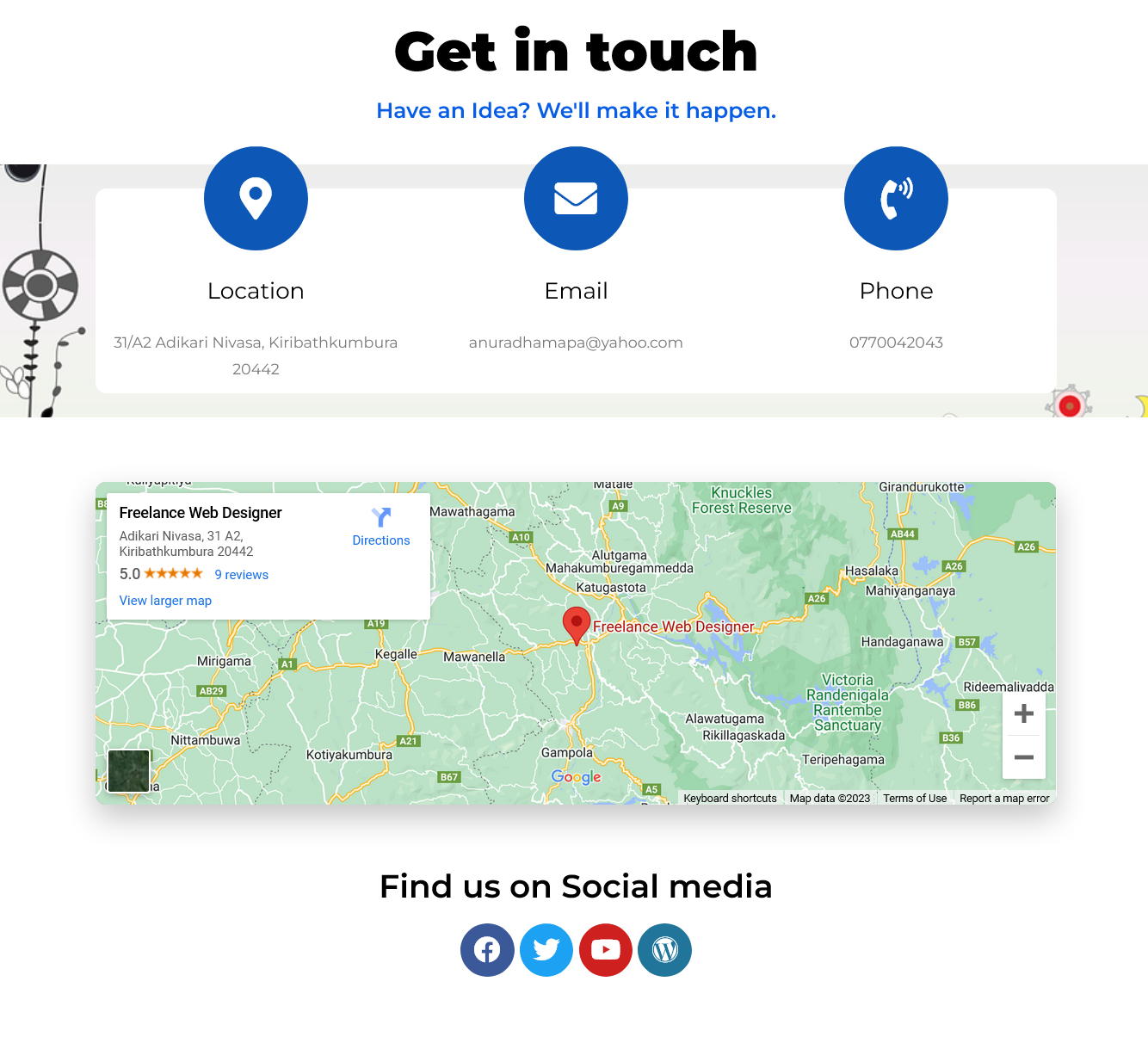Freelance Web Designer Contact Information Overlay on Google Maps

The image prominently features an overlay at the bottom displaying the contact information of a freelance web designer. The overlay is set against a Google Maps background. At the top of the overlay, a bold header, "Get in Touch," is displayed followed by a tagline in blue, "Have an idea? We'll make it happen."

The overlay contains three sections with respective icons—a pinpoint for "Location," an envelope for "Email," and a phone symbol for "Phone." The details provided are:
- **Location:** 31/A2 Adhikari Navassa, 20442
- **Email:** anuradahampy@yahoo.com
- **Phone Number:** [Phone number not provided, assumed to be there]

A white border frames the overlay, which is set against a light gray background with wallpaper designs. In the lower right corner of the overlay, there are illustrations of a red gearbox and a black-and-white life preserver with ropes hanging around it.

The detailed information includes the designation "Freelance Web Designer." A review section shows an impressive five out of five stars rating. There is also a "Directions" button that promises to provide pinpoint navigation. The map details surrounding the overlay highlight various roads leading to the specified location, marked with a red pin.

At the bottom of the overlay, social media icons indicate that the web designer can be found on Facebook, Twitter, YouTube, and one unclear network represented as "W."